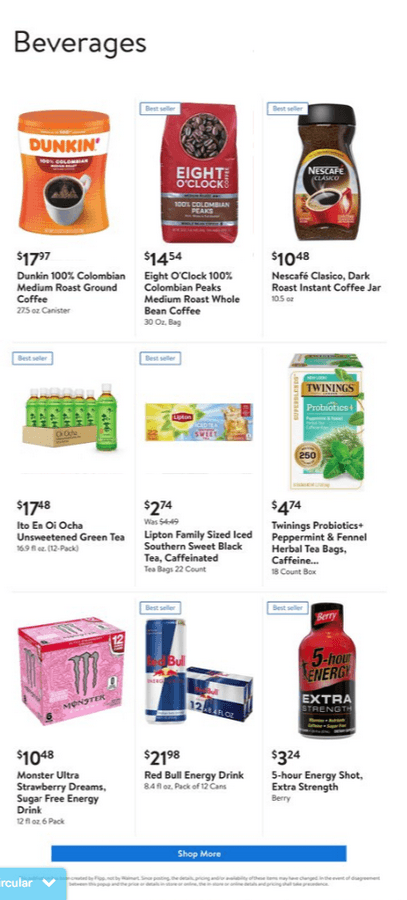This smartphone screenshot showcases a selection of nine food and grocery products available for purchase, arranged in a grid format. 

From the top left, proceeding rightward: 
1. **Dunkin' Donuts Coffee** – 100% Colombian Medium Ground Roast Coffee, priced at $17.97.
2. **8 O'Clock Coffee** – 100% Colombian Peaks Medium Roast Whole Bean Coffee, 30 oz bag, priced at $14.54.
3. **Nescafe Clasico Dark Roast Instant Coffee** – priced at $10.48.
4. **Ito En Oi Ocha Unsweetened Green Tea** – priced at $17.48.
5. **Lipton Family-Sized Iced Southern Sweet Black Tea** – Caffeinated tea bags, 22 count, priced at $2.74.
6. **Twinnings Probiotics Peppermint and Fennel Herbal Tea Bags** – Caffeine-free, priced at $4.74.
7. **Monster Ultra Strawberry Dreams Sugar-Free Energy Drink** – priced at $10.48.
8. **Red Bull Energy Drink** – priced at $21.98.
9. **5-hour Energy Shot, Extra Strength Berry** – priced at $3.24.

A blue "Shop More" button is located at the bottom of the screenshot.